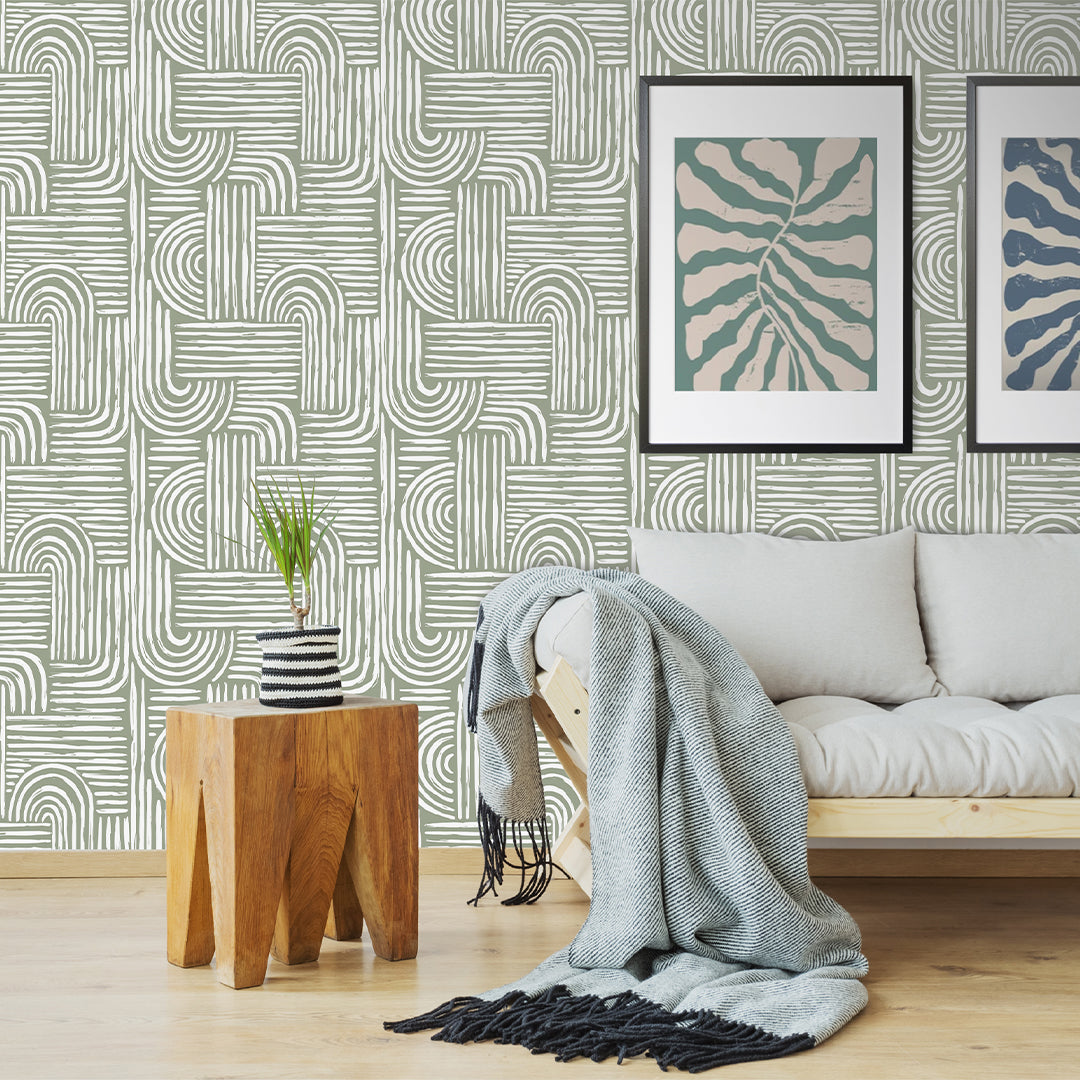This photograph showcases the interior of a meticulously designed living room, emphasizing a bright and natural ambiance. The room appears to be staged, possibly for a home decor catalog or a design portfolio. Central to the scene is a low, beige fabric sofa, exuding comfort and style, accented by a green and white twill throw blanket draped casually over its side. A small wooden table stands beside the sofa, adorned with a lush potted plant, adding a touch of greenery to the space. The walls are covered in olive-colored wallpaper featuring elegant white swirl patterns that enhance the bohemian feel of the room. Completing the artistic decor are two abstract leaf artworks that hang on the wall, adding a final touch of sophistication to this inviting interior.